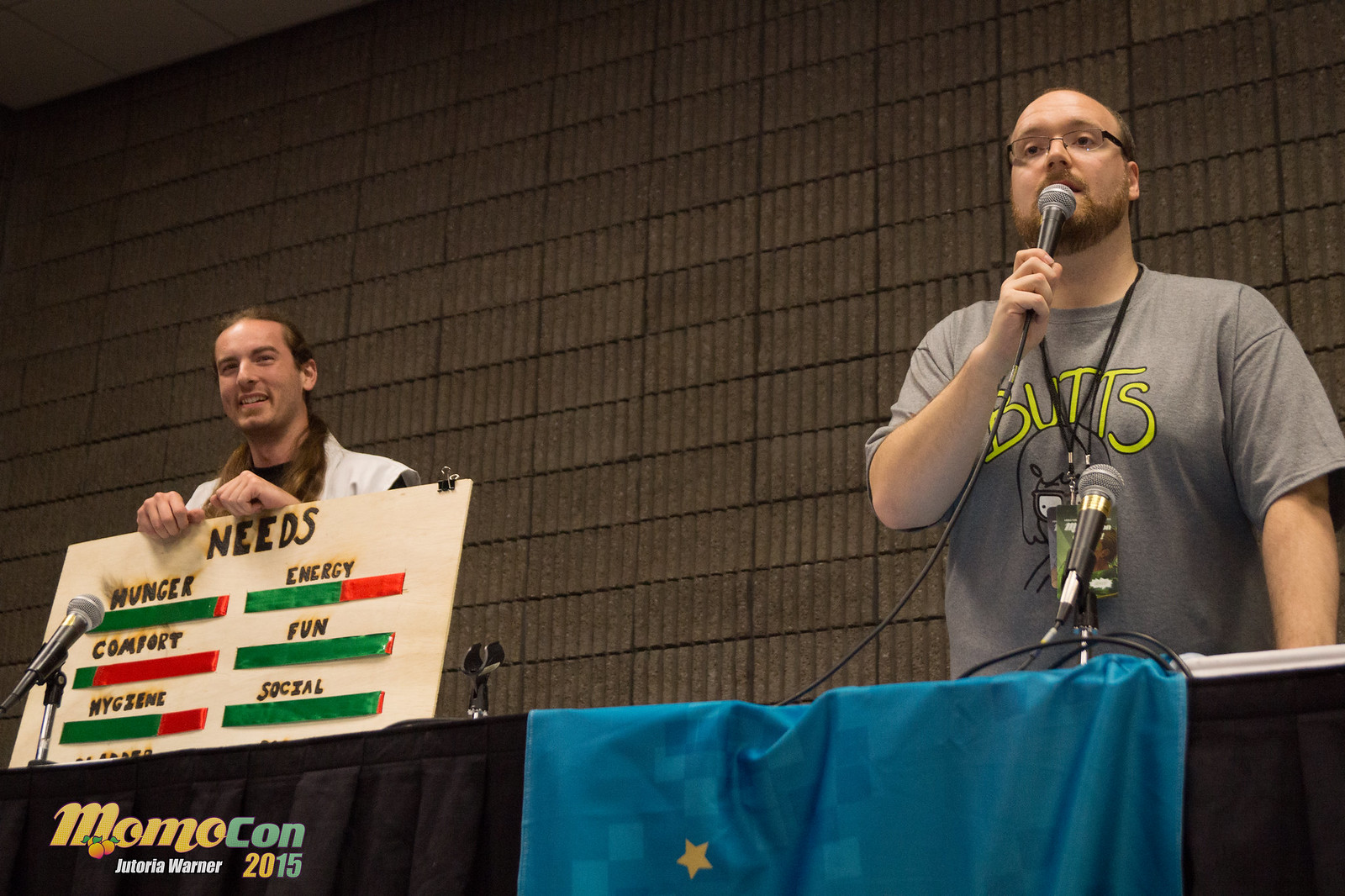The photograph depicts a scene from MomoCon Jutoria, Warner, 2015, featuring two male speakers at a convention, situated behind a desk with the perspective of the camera being below waist height. The background showcases soundproofing foam with a distinctive textured pattern resembling tiny vertical pillars stacked closely together. The speaker on the right is wearing a gray shirt with the word "Butts" spelled out in yellow text. He has glasses, a beard, and a lanyard with an ID around his neck. He is speaking into a wired microphone and there is another microphone on the table in front of him. The speaker on the left, who has long brown hair pulled back, is dressed in a white vest over a black shirt and is holding up a sign labeled "Needs." The sign displays different needs represented by bar graphs: Hunger, Energy, Comfort, Fun, Hygiene, and Social, with green segments indicating the level of need and red segments showing the unmet portions. The top needs are Hunger, Fun, and Social, followed by Energy and Hygiene in the middle, with Comfort being the least needed.